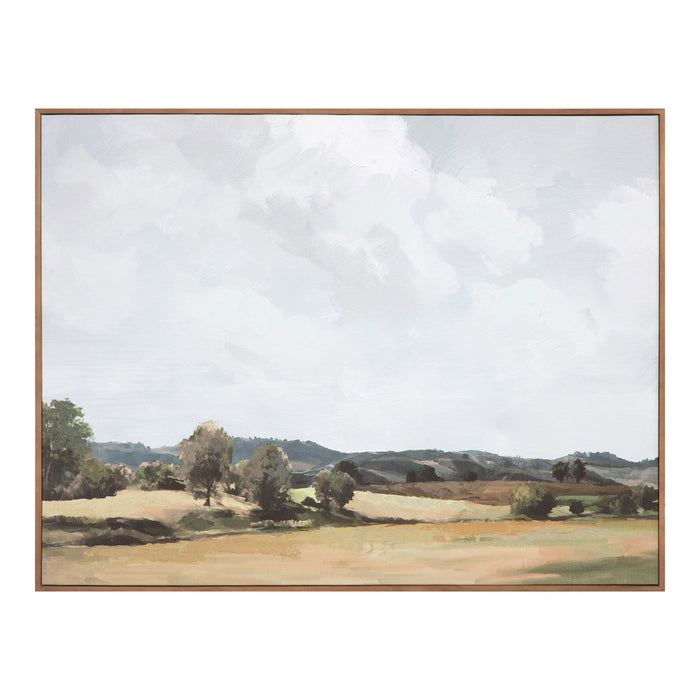The painting titled "Vast Country" depicts an expansive outdoor scene with the majority of its elements centered towards the bottom of the image. In the foreground, there's a plain brown field interspersed with sparse, gray trees and small green bushes. A slightly taller green tree is situated on the bottom left, not quite at the very edge but prominently placed. The midground is characterized by low, gray hills extending into the background, adding a sense of depth to the landscape. Towards the bottom right, there's a darker area, possibly a shadowy patch that contrasts with the muted tones of the rest of the painting. The terrain is largely level and barren, contributing to the vast, open feel of the scene.

Dominating the painting, the sky stretches across the majority of the canvas, descending past the middle of the image. It features a palette of white, blue, and some gray hues, with an abundance of cloud formations scattered throughout. The colors are muted, giving the painting a subdued, almost melancholic atmosphere. The lack of bright colors and detailed imagery further enhances the serene and expansive nature of the countryside depicted in the artwork.